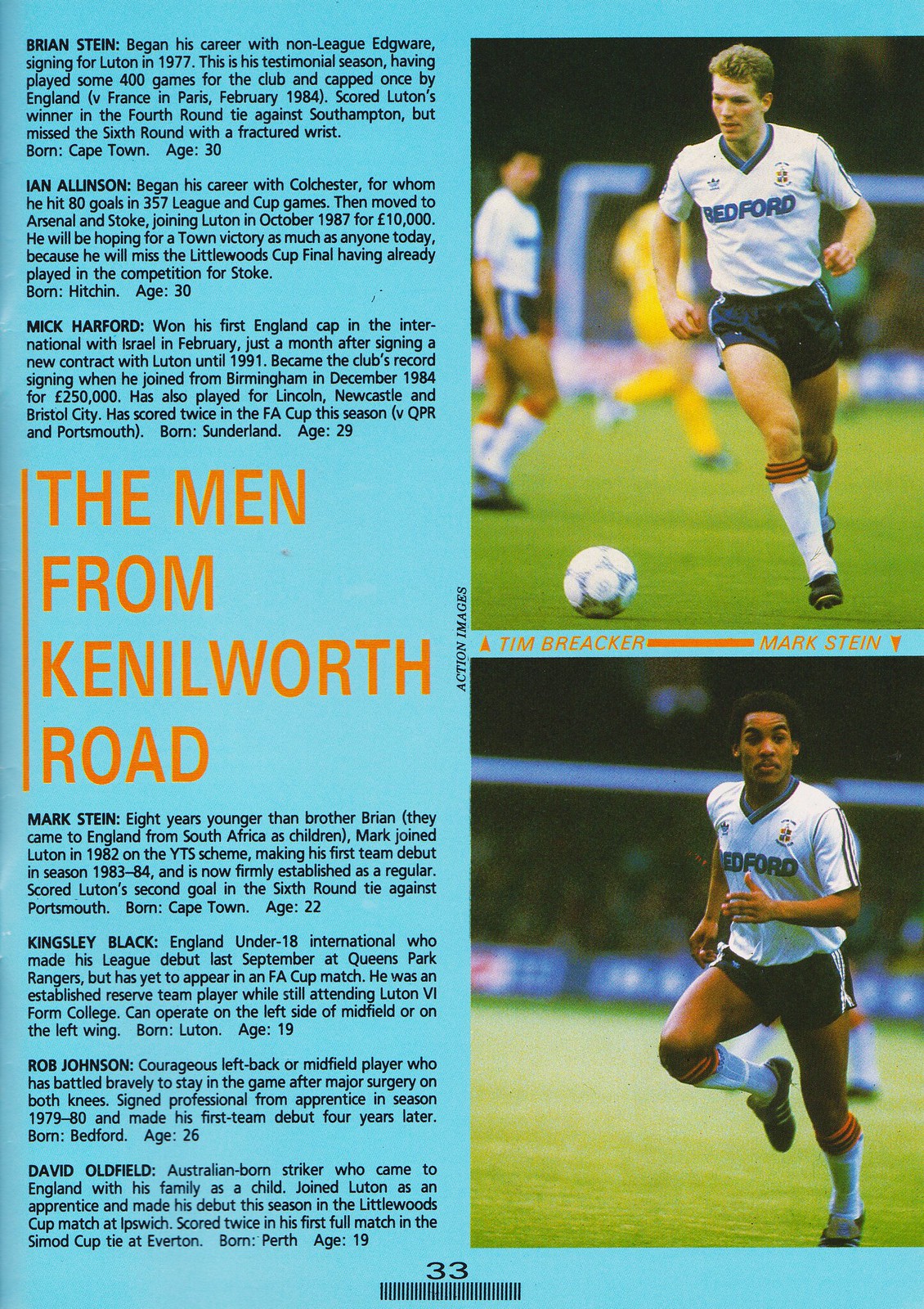The image appears to be a vintage page from a soccer program, designed on a blue piece of paper and measuring about six inches tall by four inches wide. The page is divided into two distinct sections. On the left side, black-printed text provides short biographies of several team members, including Brian Stein, Ian Allenson, Nick Harford, Mark Stein, Kingsley Black, Rob Johnson, and David Oldfield. These biographies detail each player's background, age, and other relevant information. Down the center, an orange vertical line separates the text from the right-hand side. At the top of the right-hand side, an orange label reads "The Men from Kenilworth Road," referring to the team's association with Kenilworth Road. Below this, the section is split into two images, one above the other. The top photograph features Tim Breaker, a young white man with short brown hair, dressed in a white and blue jersey and black shorts, running towards a soccer ball on the grass. Behind him, other players are visible in a non-active stance, suggesting a practice session. The bottom photograph shows Mark Stein, a young black man in a similar jersey and shorts, running in a different direction as if positioning to receive a pass. Both players are depicted on a football pitch, contributing to the program's detailed presentation of the team's roster and activities.